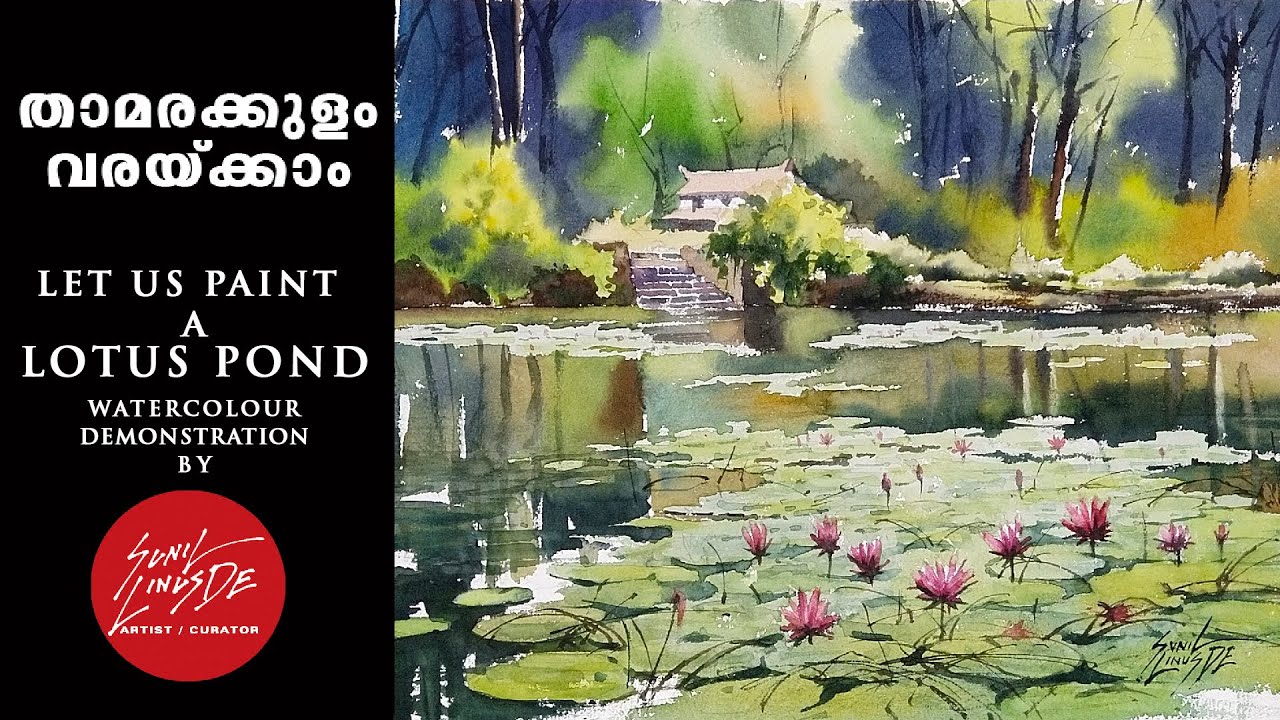The horizontally aligned rectangular image is divided into two distinct sections. The left side features a thick black background adorned with two rows of white symbols resembling letters at the top. Beneath these symbols, white text reads, "Let us paint a lotus pond. Watercolor demonstration by," followed by a red circle containing white letters that spell out, "Sunil Lindsay, artist/curator." On the right side, the image transitions into a detailed painting of a serene pond abundant with green lily pads and pink flowers. The pond reflects its surroundings, which include green trees with brown and black trunks, some appearing snow-dusted. In the background, partially obscured by trees, stands a two-story house with a tan or white exterior and what appears to be a blue or bluish-black sky above. This idyllic setting is further complemented by purple and gray steps leading down towards the water. Finally, the bottom right corner of the painting features the text, "Sonny Linus Day," also in black.